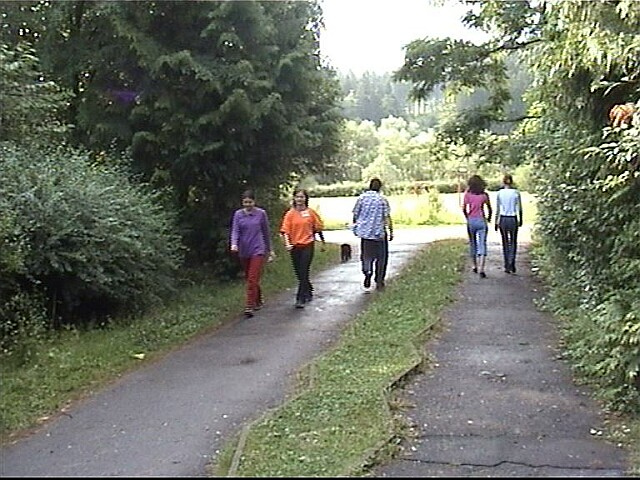The image captures a serene, green city park with a dual-paved walking trail separated by a grassy median. Flanking the pathway, lush vegetation of thick trees, vines, and shrubs envelops the scene. The trail appears to be maintained, though the grass in the median looks slightly overgrown. The path leads to another trail, beyond which a glimmer of sunlight suggests the presence of a lake or river, adding to the tranquil setting. 

The scene is populated with several people: two young women in a pink and an orange shirt walk away from the camera on the right path, while a young man in black pants and a maroon shirt does the same on the left. Another pair, consisting of a girl in a purple shirt and another in a checkered white and blue shirt with denim jeans, walks towards the camera on the left side, accompanied by a small dog. The cracked pavement and the slightly grainy resolution hint that this might be a screenshot from a video. The overall feel of the image is peaceful and inviting, perfect for a walk away from the hustle and bustle.